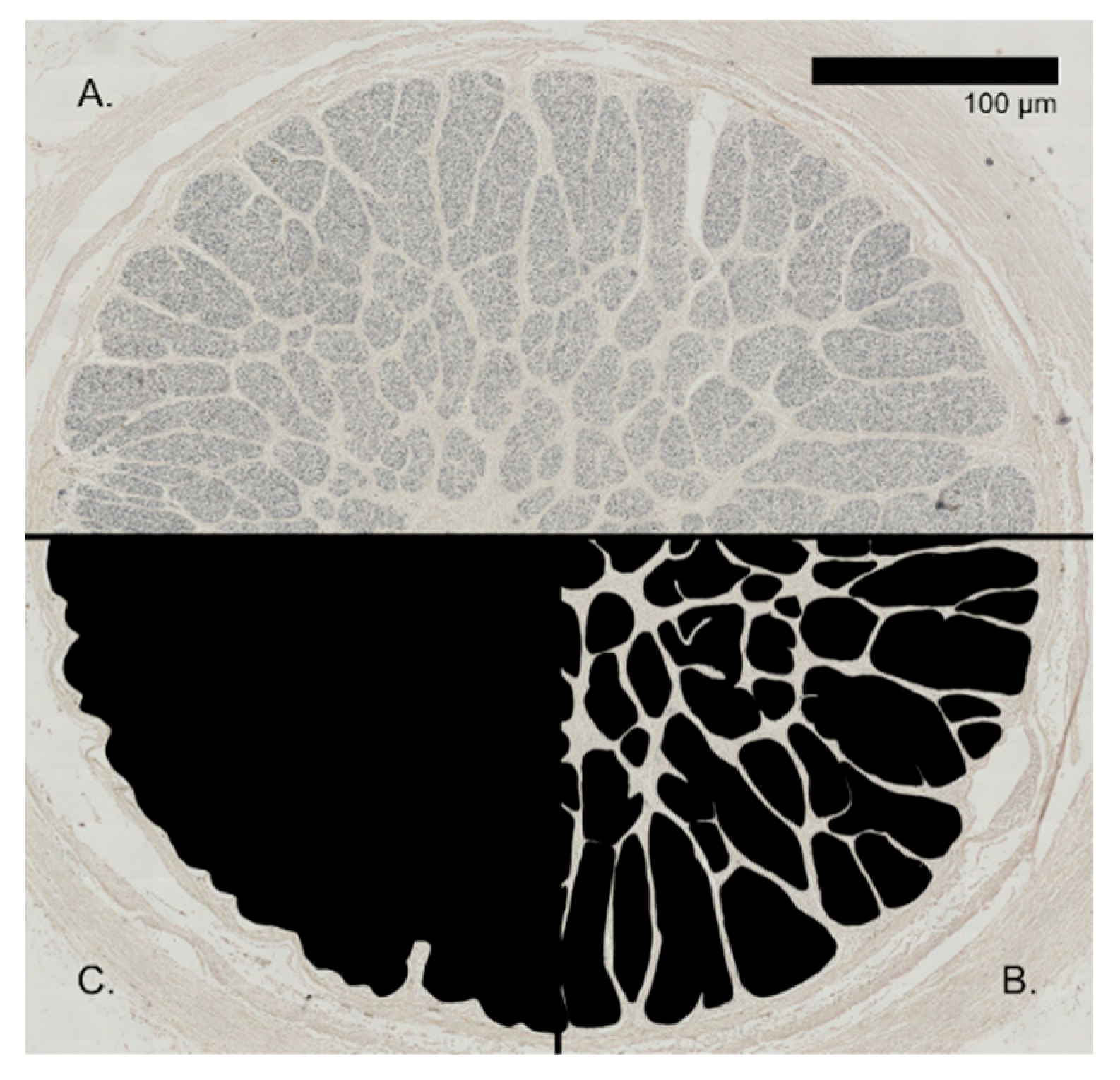The detailed black, white, and gray illustration appears to be a biological diagram, possibly of an optic nerve, displayed in a circular format. The image is divided into three distinct sections. The top semi-circle, labeled "A" on the top-left corner, is filled with light gray, intricate vein-like patterns. A horizontal line runs through the center of the circle, demarcating the top part from the bottom. Below this line, the bottom part is vertically divided into two segments: the left side, labeled "C" at the bottom left, is pitch black with jagged edges, while the right side, labeled "B" at the bottom right, features solid black vein-like patterns against a lighter gray background, resembling spots. At the very top-right corner of the image, a black bar labeled "100UM" indicates the scale of the diagram. The entire image has a faint light gray circular border, suggesting the illustration represents a single organism or anatomical structure.